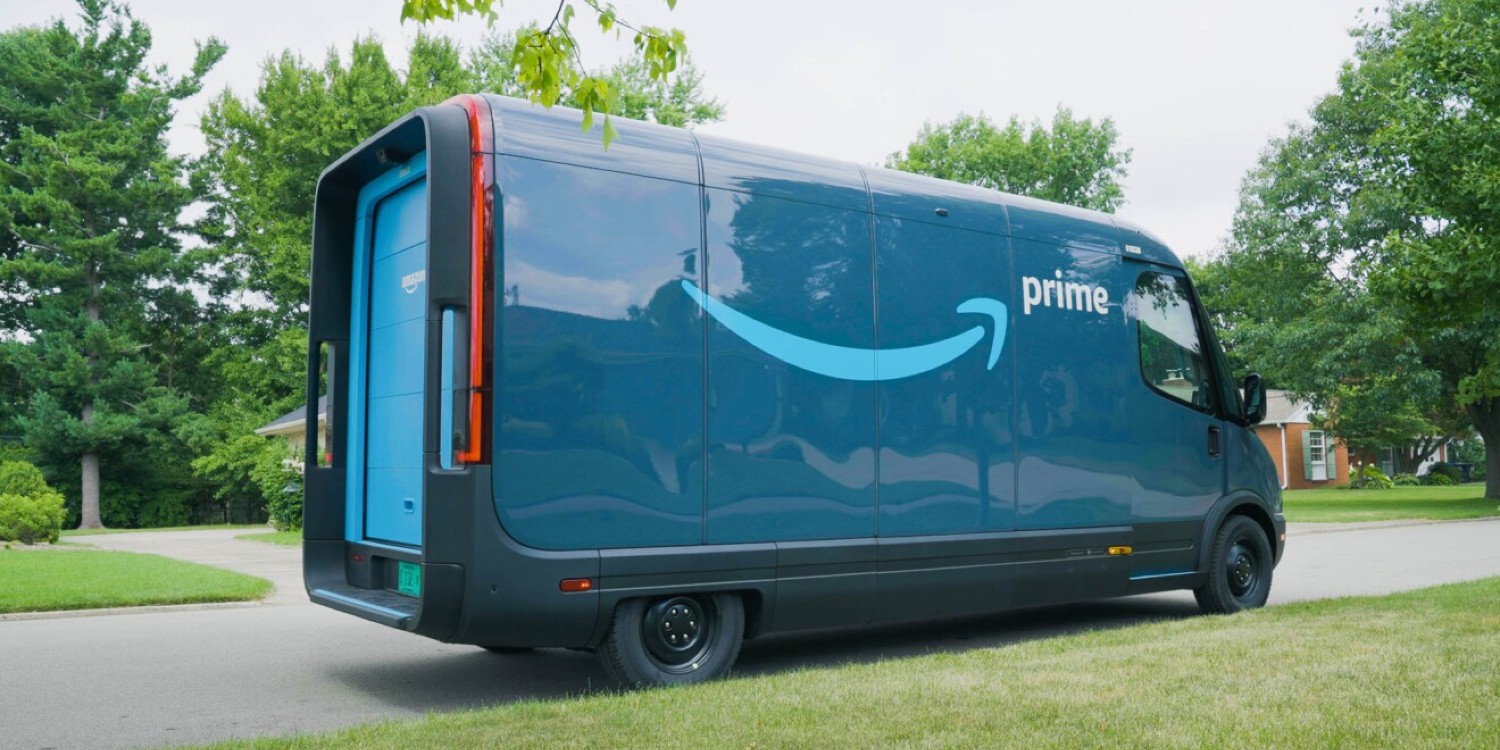In this daytime photograph, a large Amazon Prime delivery van is prominently featured, parked on a gray concrete driveway in a residential neighborhood. The van is painted in hues of royal and light blue, showcasing the iconic white Amazon smile logo and the word "Prime." The back door of the van also bears the Amazon name in white letters. The van has black wheels, and details such as bolt rivets are visible on the tires. The vehicle's side also includes orange lights, and a teal license plate is noticeable.

Surrounding the van, the residential backdrop includes green grass of varying lengths and several mature trees with lush foliage. An orange brick house with green shutters is visible in the distance, adding a homely charm to the scene. The sky above is overcast, casting a soft, diffused light across the landscape, with light reflections visible on the van's surface. At the top of the image, green leaves from the trees slightly frame the scene. The photograph is crisp and clear, capturing intricate details and providing a vivid portrayal of suburban tranquility interspersed with modern logistics.